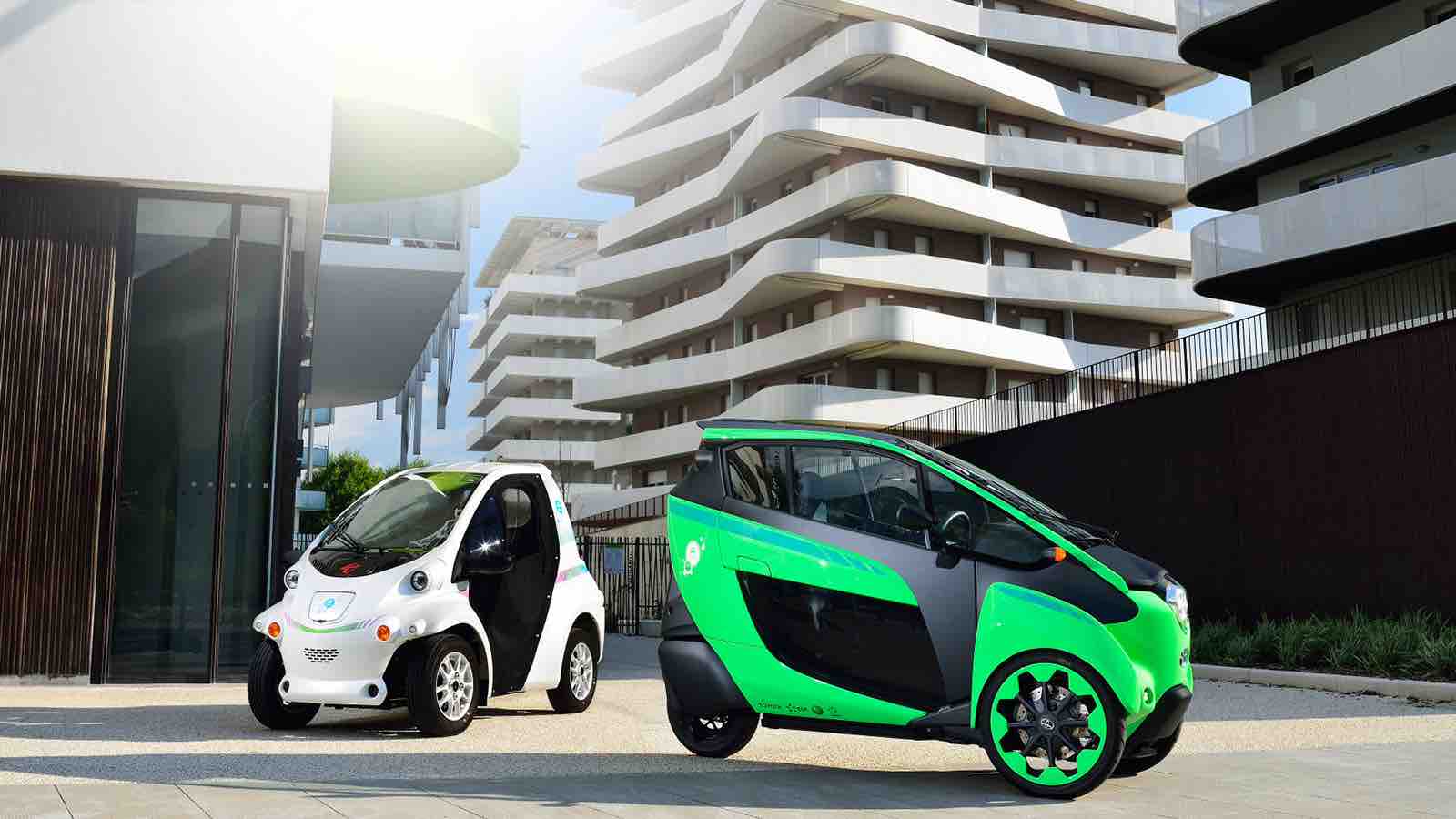This image depicts two futuristic electric cars set against a backdrop of modern, high-rise buildings. The cars, resembling compact smart cars, are positioned on a street-like surface. The vehicle on the left is white with four small wheels and no doors, while the one on the right is green and black, featuring three wheels—two at the front and one at the back—and equipped with doors. The architecture in the background includes three distinctive high-rise buildings, each about 8 to 9 stories tall, featuring an intricate offset design with square, plate-like structures jutting out in a staggered fashion. To the left, another building stands with an open, circular entryway, and a black fence is visible in the right foreground. The entire scene evokes a futuristic urban landscape, possibly in a city known for its avant-garde architectural styles, such as Singapore or Dubai.